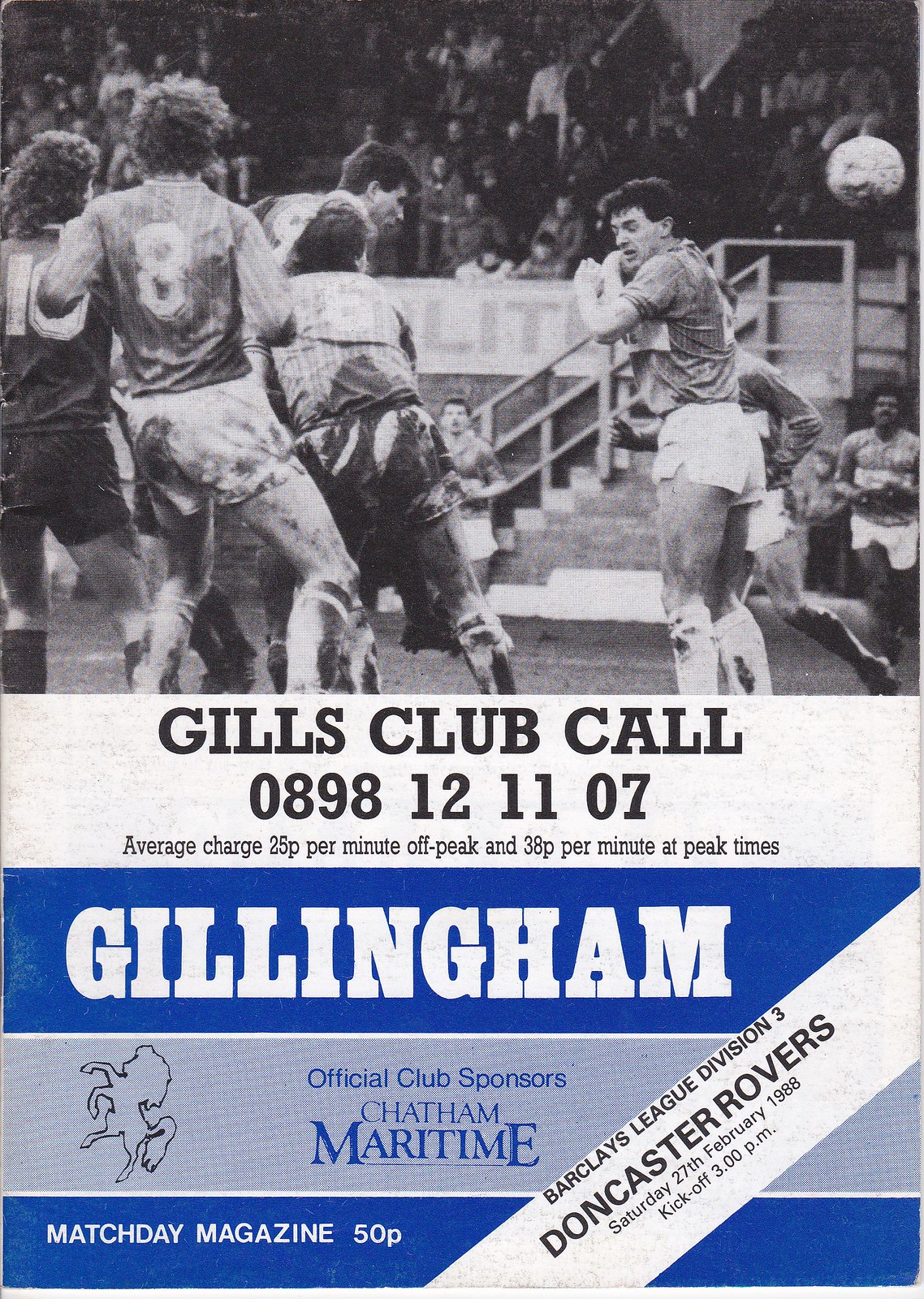This is the cover of a match day program for a soccer game from Gillingham FC, dating back to Saturday, February 27, 1988. Priced at 50 pence, it marks a clash against Doncaster Rovers in the Barclays League Division 3, with a kickoff scheduled for 3 p.m. The sponsorship by Chatham Maritime is prominently mentioned. 

The cover features a dynamic black-and-white photo capturing an intense moment on the field. Centered around a soccer ball suspended mid-air, several players, clad in numbered shirts and shorts, are fiercely competing. One player standing to the right appears upset or uncomfortable, while a cluster of players to his left wrestle for positioning, their determination vividly shown by their tussle and dirt-streaked attire. The background shows spectators in the stands, adding a sense of anticipation and excitement.

Above the image, contact details for the Gills Club are provided: 0898 121107, with calls costing 25 pence per minute off-peak and 30 pence per minute at peak times. This action-packed cover effectively conveys the fervor and competitiveness associated with the game, urging fans to relish in the thrill of the sport.